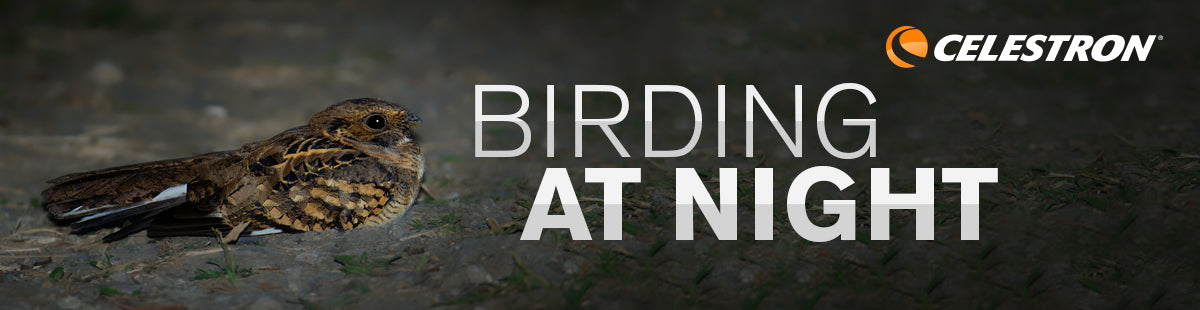The image is a rectangular advertisement measuring approximately 11 to 12 inches wide and 5 to 6 inches tall, promoting Celestron's "Birding at Night." The text "birding" is presented in a thin, white font, while "at night" is in a chunkier, more dramatic font. On the left side of the ad, there's a detailed image of a small bird at rest on the ground, its long wings displaying various shades of brown with light brown spots at the center of its body. The bird's small head and barely visible beak add to the nocturnal mystique. The background is blurred, enhancing the nighttime setting. To the right of the image, the text "Celestron" appears along with the company's orange emblem. This ad, which could serve as a web banner or poster, has a striking and dramatic visual appeal, making it effective for promoting birdwatching activities at night.